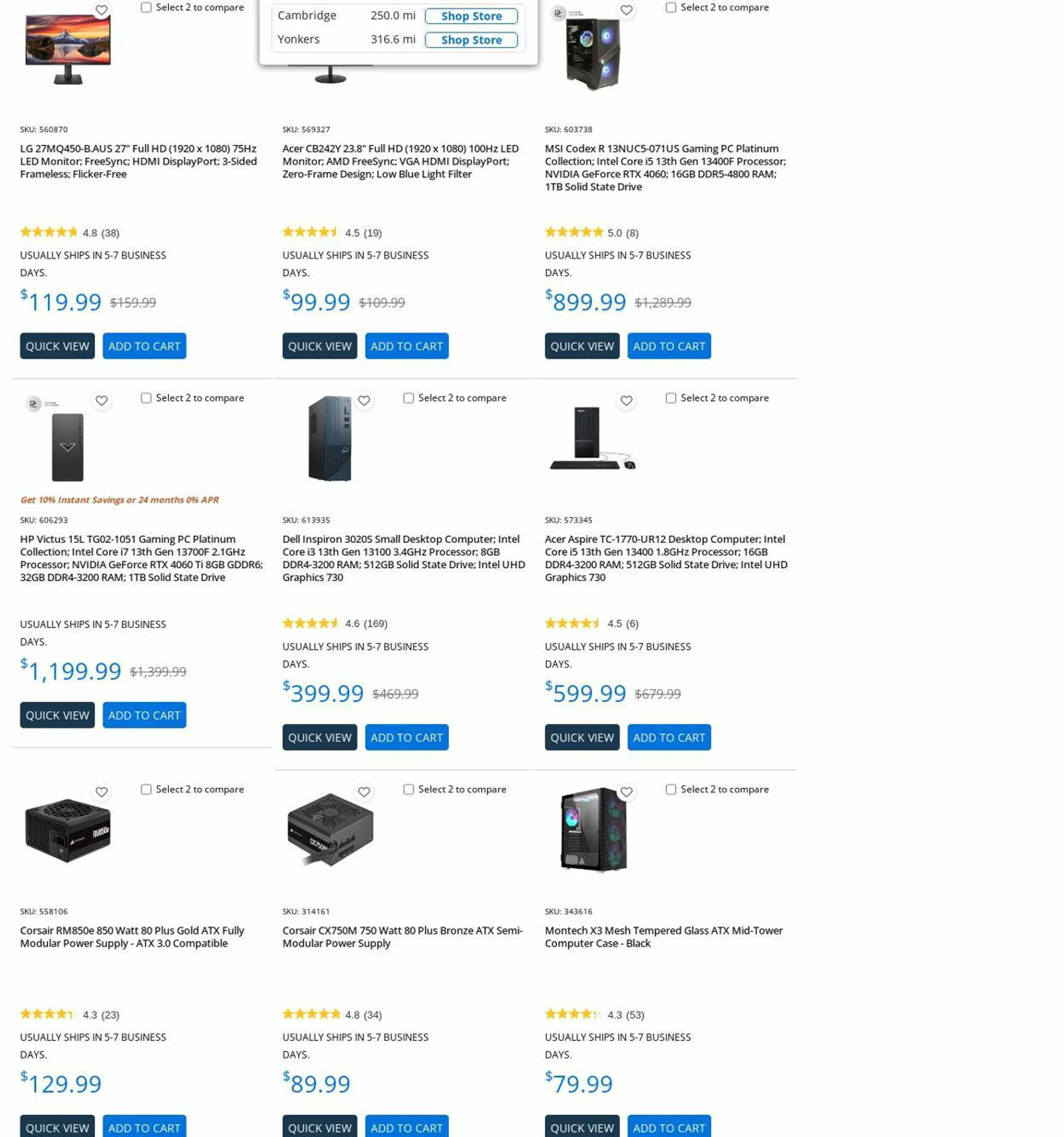The image depicts a screenshot from an online store specializing in computer hardware and electronics. It showcases a grid layout featuring nine thumbnails, organized in a 3x3 format.

- **Top Row:**
  - The first item in the top left is a computer screen priced at $119.99. The accompanying text is too small to decipher.
  - The middle thumbnail is partially cut off, but the item is listed at $99.99.
  - The item on the top right appears to be a desktop computer priced at $899.99.

- **Middle Row:**
  - The first item on the left is another desktop computer, priced at $1,199.99.
  - The middle item also seems to be a desktop computer, this one priced at $399.99 and appears to be a Dell model.
  - On the right, the thumbnail shows a desktop computer along with a mouse and keyboard, priced at $599.99.

- **Bottom Row:**
  - The first item on the bottom left looks like a power supply unit, priced at $129.99.
  - The middle thumbnail displays another power supply unit, priced at $89.99.
  - The last item on the bottom right appears to be a desktop computer case, priced at $79.99.

Each thumbnail includes product images and prices, even though some product details are either too small to read or partly cut off.